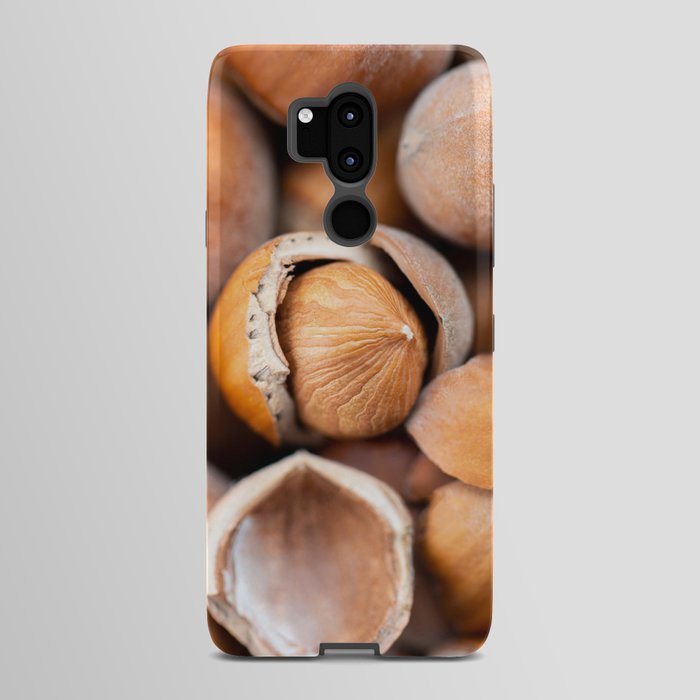The image depicts the back of a smartphone cover adorned with a detailed illustration of hazelnuts or filberts. In the center of the design, a prominent brown nut with a distinctive white dot at its tip appears nestled inside a cracked shell, forming a bowl-like shape with a white edge. This central nut features fine lines radiating from left to right, converging towards a point. Below and towards the left, an out-of-focus open nut shell with a white rim and a brown interior is visible. In the upper right corner, an intact yellowish hazelnut speckled with white dots stands out. The smartphone camera is situated towards the top-center of the cover, comprising a black circle at its base with a black oval above it, and a protruding rectangular component with a white square on its top left. The overall background of the cover features more hazelnuts in varying shades from light whitish to brown, some appearing sharper than others, adding depth and intricacy to the image.